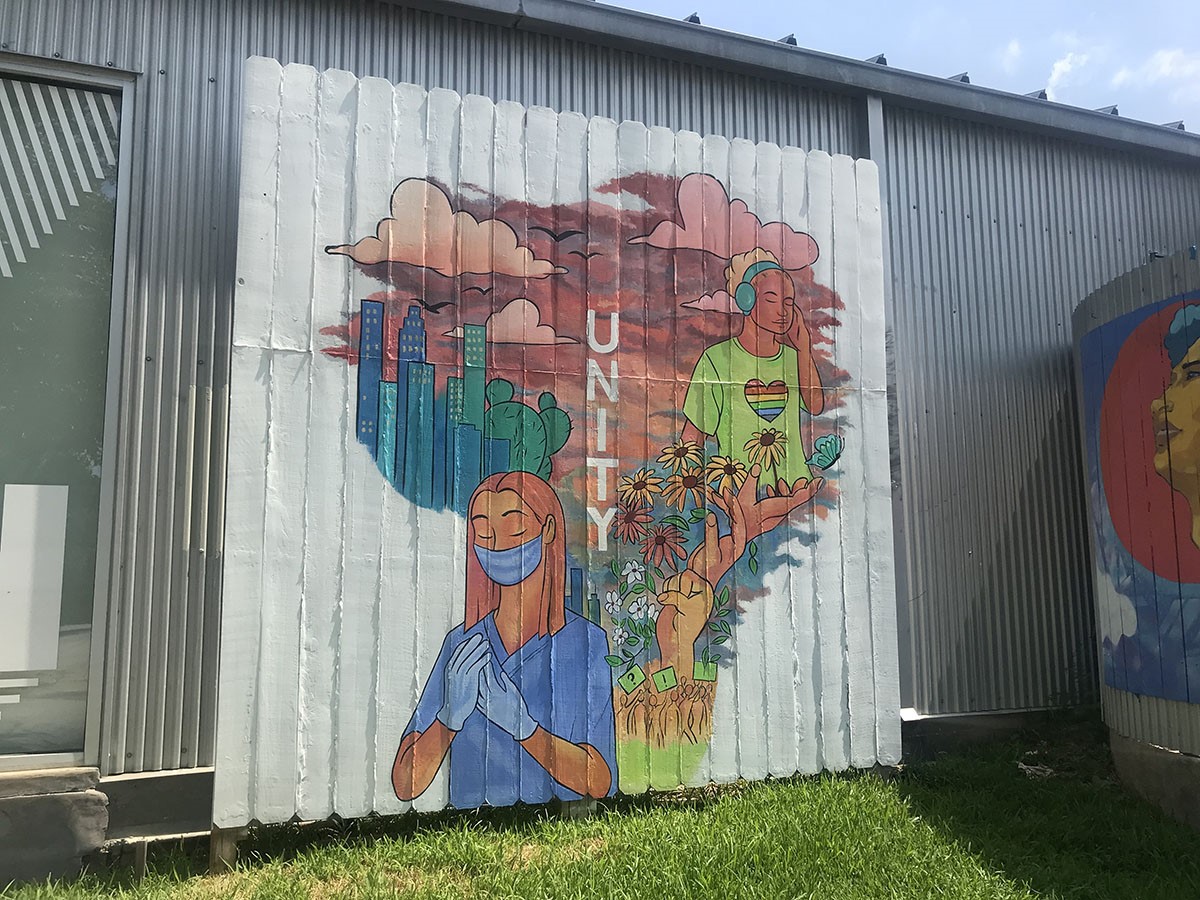The image depicts a vibrant piece of graffiti art, spanning a 7-foot section of white picket fence, set against a corrugated metal wall. The scene is viewed from a slight angle, with the left side appearing closer than the right. Intricately detailed, the artwork features dynamic elements that tell a compelling narrative. 

At the bottom left, near the grassy ground, stands a nurse in scrubs, donning a mask and blue gloves. Adjacent to her, a trio of hands emerges from a crowd, each grasping vibrant flowers, symbolizing unity and hope. To the upper right, a black woman, distinguished by her green shirt adorned with a heart and rainbow design, wears teal headphones, striking a powerful pose. 

The backdrop of the piece is a striking gradient sky, shifting from dark to light red, punctuated by dark red, orange, and dark pink clouds. On the left side, blue and green skyscrapers rise, adding an urban touch to the composition. Additionally, there's a unique element: a cityscape with a cactus, juxtaposing nature and urban life. The artwork's setting on the fence imparts a communal and accessible feel, merging personal expression with public space.